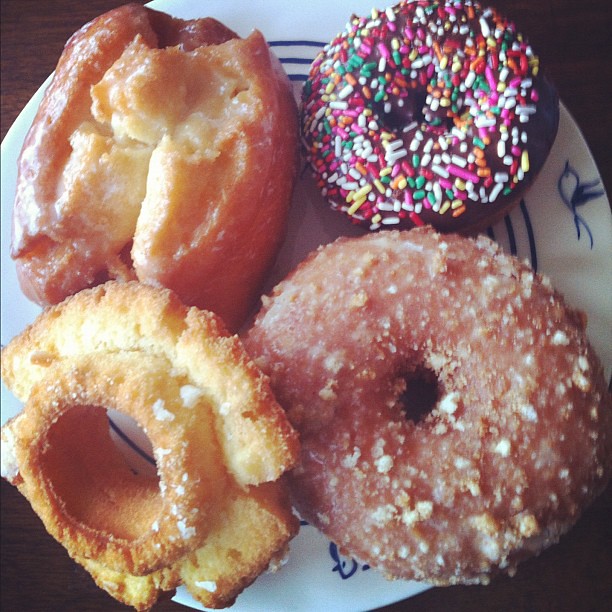This close-up photograph, taken from above, captures four distinct donuts on a small, white porcelain plate adorned with three blue lines and hand-drawn bird details around its edge. The donuts fill the plate entirely, slightly extending over its edges. In the upper left is an old-fashioned, rectangular bar-shaped donut, roughly the size of a wallet. The upper right features a traditional round donut with a nearly closed center, topped with chocolate glaze and colorful sprinkles in white, purple, light blue, green, pink, yellow, and red. The lower left holds a plain old-fashioned donut, showcasing its characteristic flat sides and break marks. Lastly, the bottom right displays a slightly larger standard donut with a more matte glaze, possibly maple. The scene is set against a wooden surface, enhancing the rustic charm of this delectable assortment.